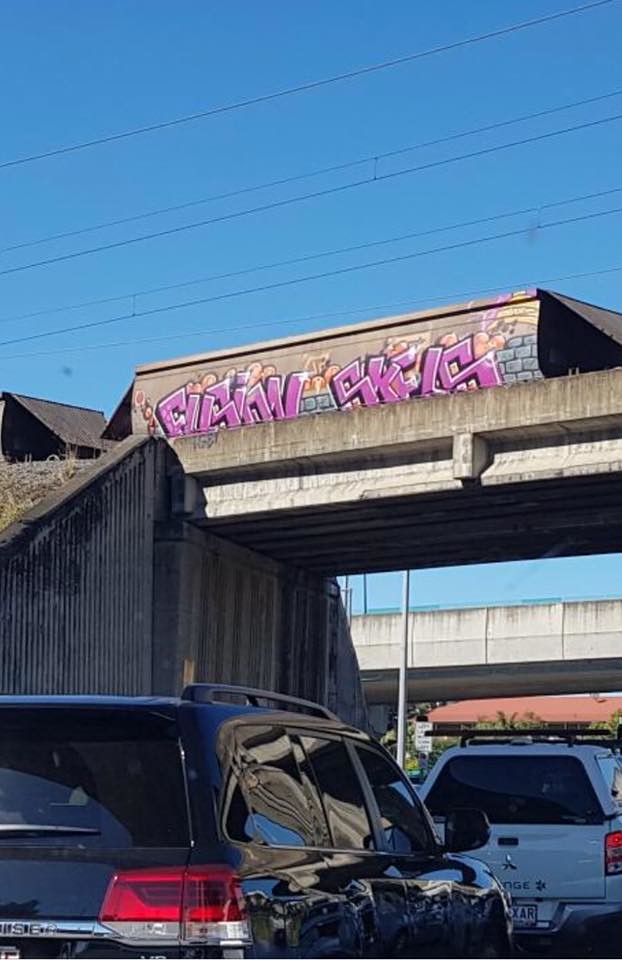The image captures a clear, sunny day with a bright blue sky. Central to the scene, two vehicles are driving under a narrow bridge or overpass, which could be part of a walkway. The vehicle in front is a white, smaller truck with a canopy and a roof rack, while the vehicle behind it is a shiny black SUV also equipped with a roof rack. Only the rear and partial sides of these cars are visible due to the angle of the photograph. Above the overpass is a graffiti artwork consisting of two words in pink lettering outlined in black. In the background, additional electrical wires and a house on the left are visible, as well as another overpass farther ahead.